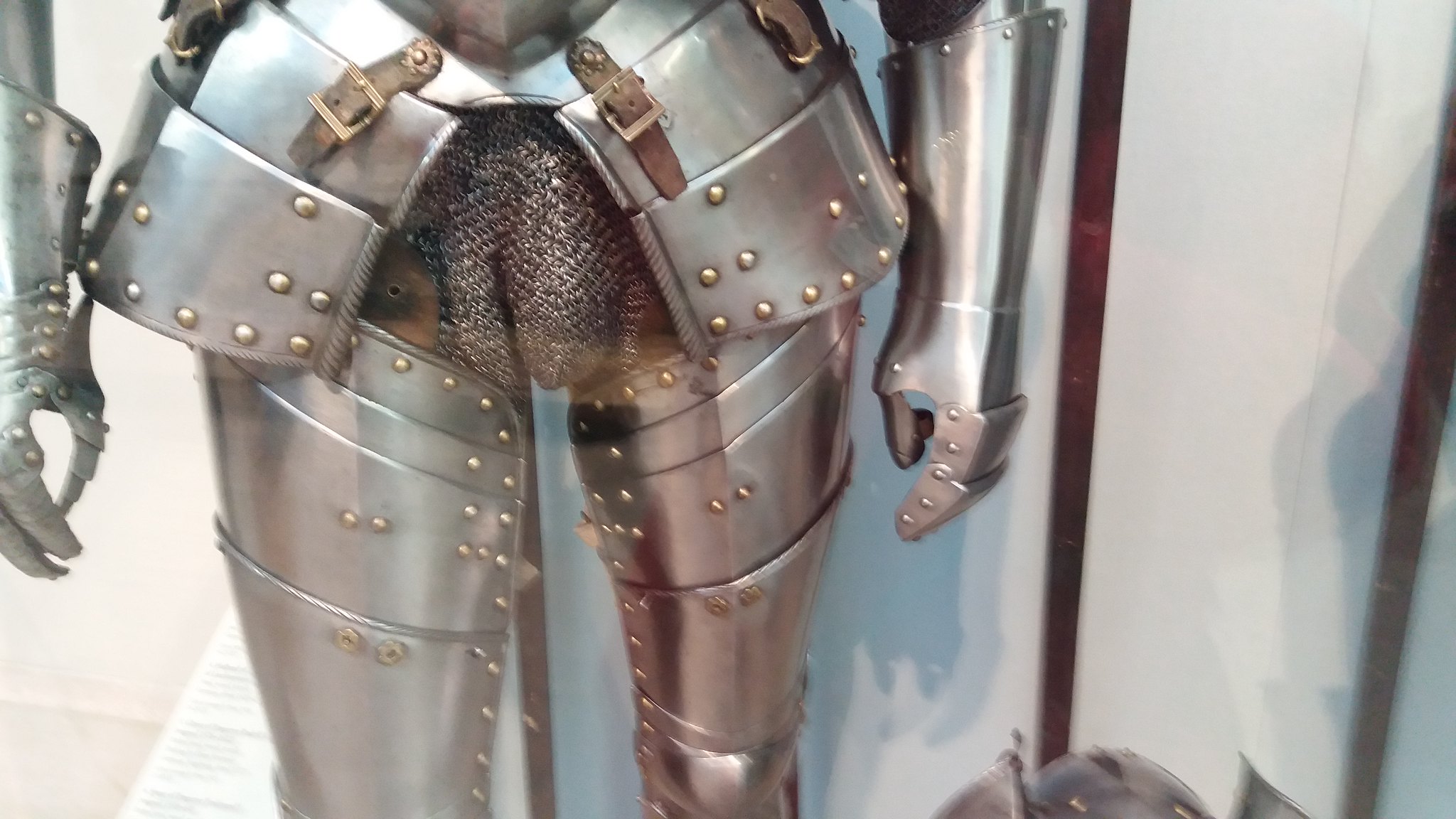The image showcases a close-up, slightly blurry shot of the lower section of a suit of armor, concentrating on the groin and hips area. The unpainted stainless metal plates are riveted together with small tacks, giving it a historical yet unfinished look. Below the waist, the armor is segmented and covers the calves and thighs, with interconnected plates. Notably, there is a small gap in the skirt revealing tightly fitted chainmail underneath, filling any potential gaps for protection. The surroundings hint at a studio setup with a grayish-silver backdrop and white shading, with hints of items like brown sticks possibly used for display or support. The armor itself appears vacant, without any person inside, adding to the sense that this might be a reproduction or new model intended for display purposes.